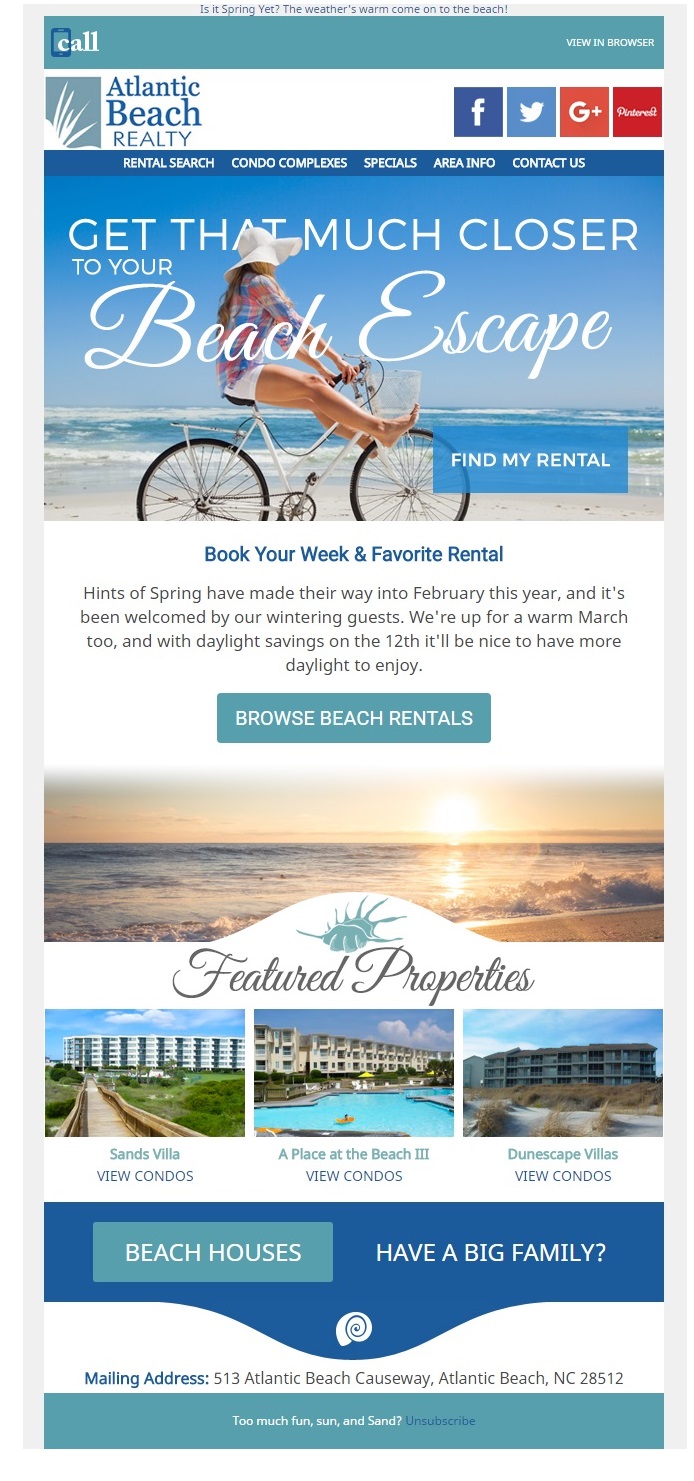This is a detailed descriptive caption for the given image:

The screenshot showcases the homepage of the Atlantic Beach Royalty website, a real estate agency. Dominating the top section is an inviting image of a woman joyfully riding a bicycle along a beach under a clear blue sky. She is dressed in white shorts, a colorful checkered shirt, and a wide brimmed white hat. Capturing a carefree holiday spirit, her feet are lifted off the pedals as she glides along. Overlaid on this image is the enticing text, "Get that much closer to your beach escape," accompanied by a blue button with white text that reads, "Find my rental." 

Beneath this main image, there is a call-to-action slogan in black text that says, "Book your weekend favorite rental." Further down, users are prompted to browse available beach rentals via an additional button. Below this section, there is a banner featuring three images of different properties labeled as "featured properties." These include Sands Villa, A Place at the Beach 3, and Dunescape Villas, all of which are condominium options.